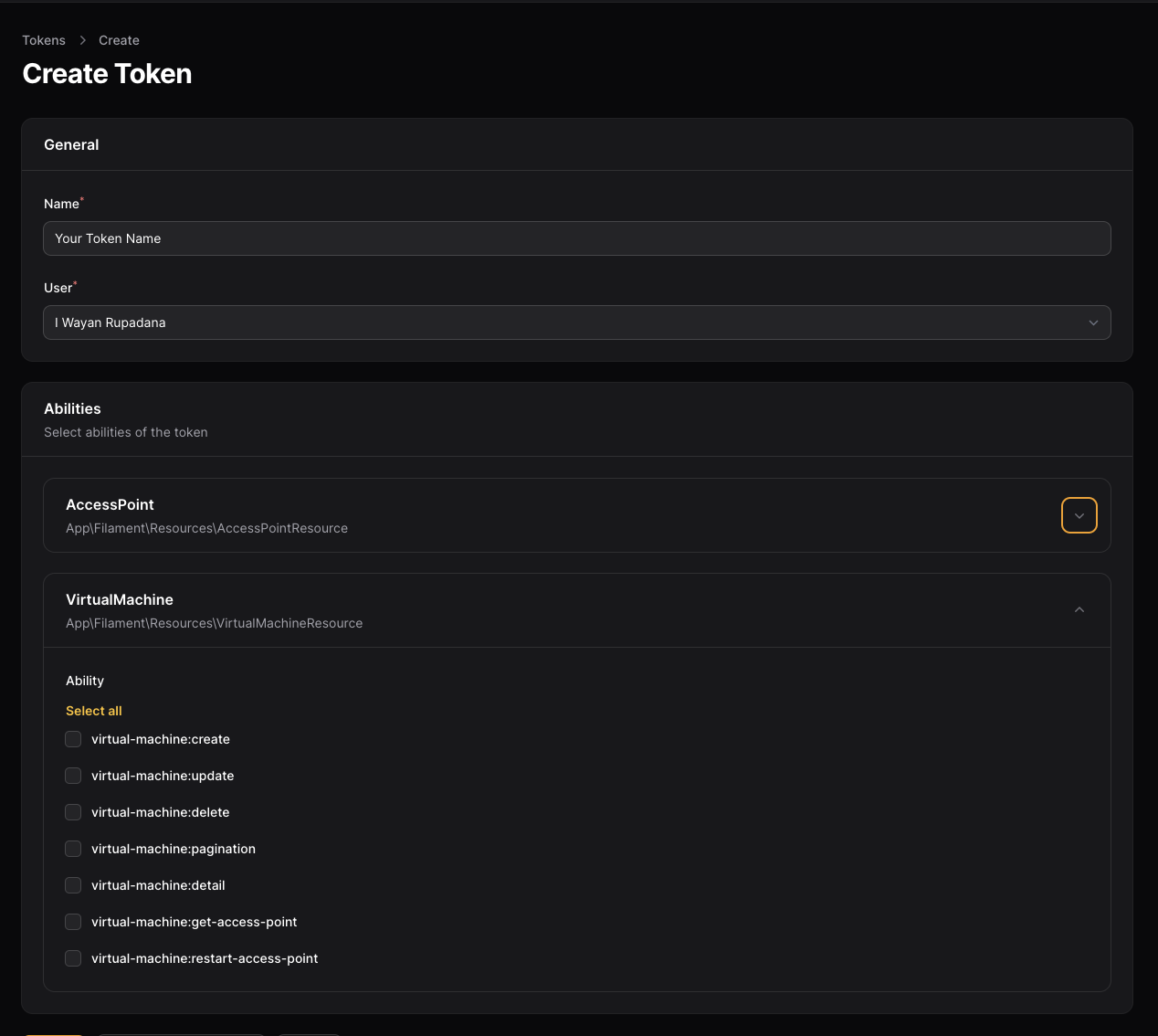The image features a user interface with a black background. At the top, it displays the heading "Tokens Create." Below this heading, in large bold white letters, it prominently reads "Create Token." Underneath, there’s a section labeled "General." Within this section:

- There is a field labeled "Name," accompanied by a text box that reads "Your token name."
- Next, there’s a field labeled "User," along with a text box below it containing the name "I Wayan Rupadana."
- Following this, there is a section for "Abilities," where users can select abilities for the token. Below this section:
  - There is a box labeled "Access Point App/Filament/Resources/Access Point Resource," highlighted with an orange border and accompanied by a drop-down menu.
  - Another option follows, marked "Virtual Machine App/Filament/Resources/Virtual Machine Resource."

Additionally, there are options related to abilities:
- In bold orange text, there is an "Ability" header followed by the option "Select All."
- Below this, options listed include "Virtual-Machine Create" and "Virtual/Machine Update."